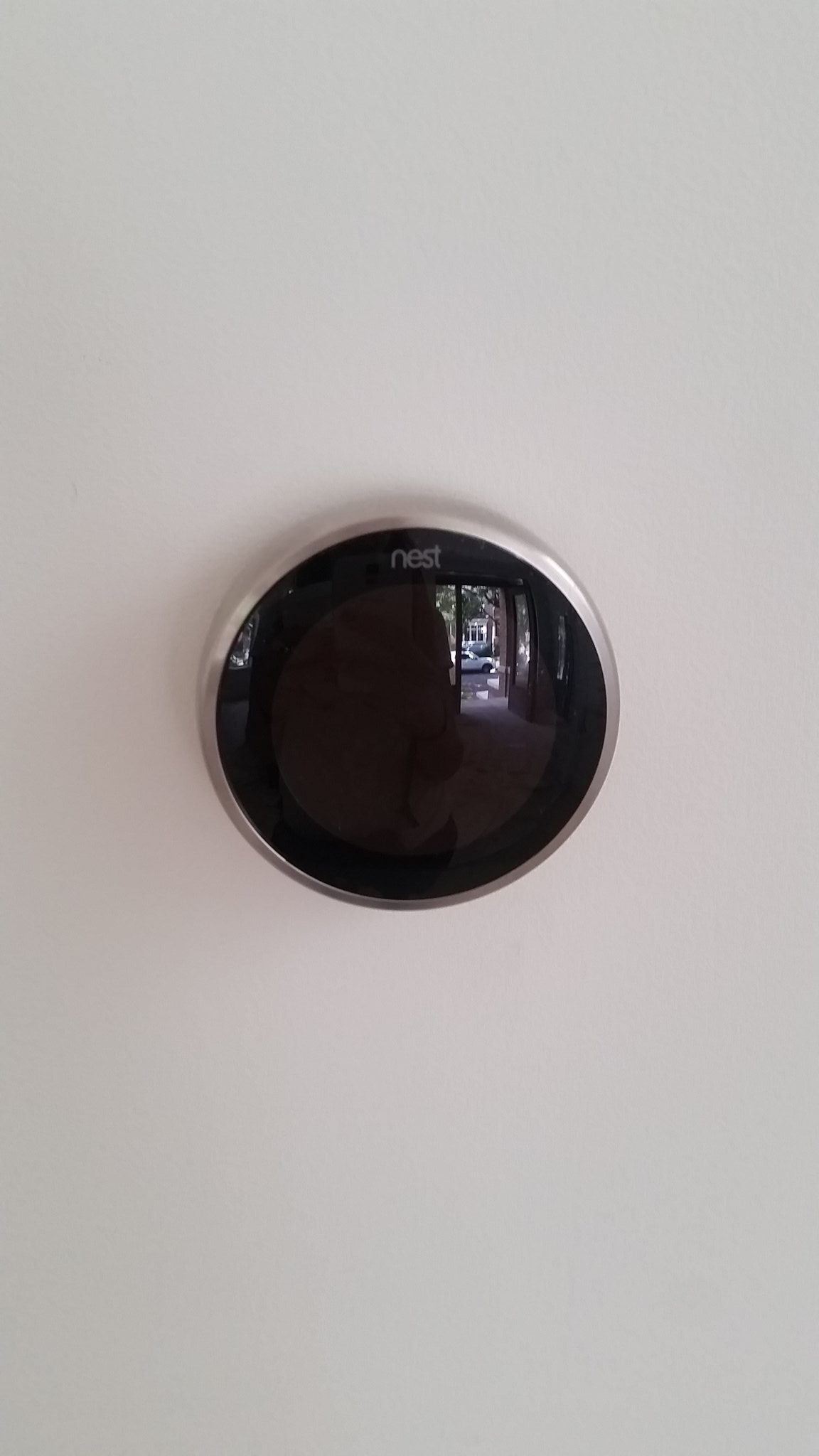This image captures a Nest security camera mounted on a white wall. The camera is spherical with a glossy, black, and highly reflective globe-like covering and features a silver rounded edge. The word "nest" is displayed in lowercase, white lettering at the top of the camera. Through the reflection on the camera's surface, a partially open door can be seen, revealing an outdoor scene. In the background of this reflection, there is a street in daylight with a white car parked and a house visible. Additionally, some dark shapes are observed along the camera's glass, adding to the detailed reflection.